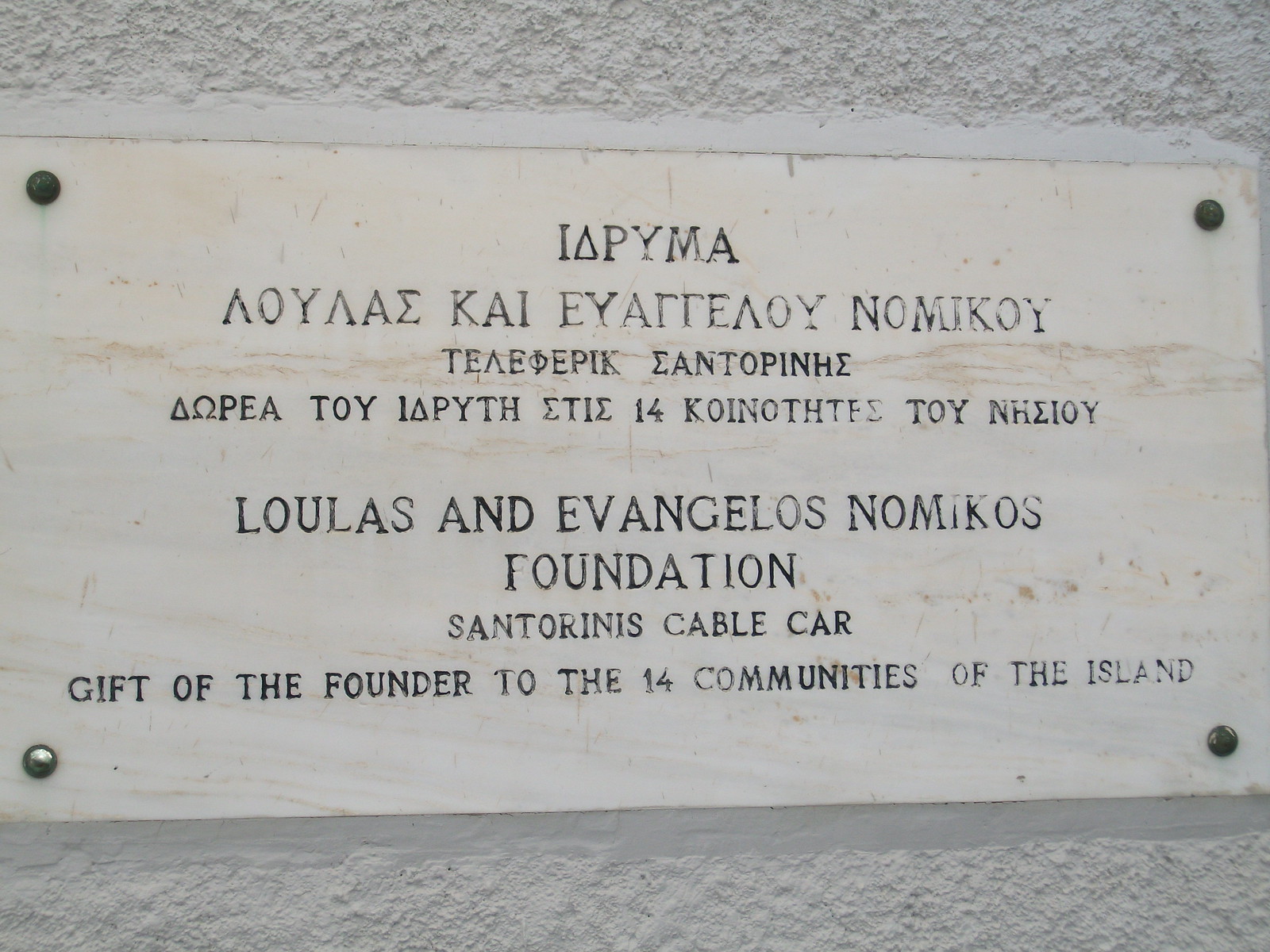The image depicts a white, rectangular plaque that appears to be riveted onto a white stone wall, likely the side of a building. The plaque is secured with four rivets, one at each corner. The top half of the plaque features text etched in Greek, while the bottom half contains an English inscription. The English text reads: "Lulus and Evangelos Nomikos Foundation Santorini's Cable Car, gift of the founder to the 14 communities of the island." The plaque seems to be crafted from either white marble or a white metal, and the wall it is attached to has a rough, block-like texture. The setting is inferred to be Santorini, Greece, given the bilingual nature of the inscription and the reference to the island.